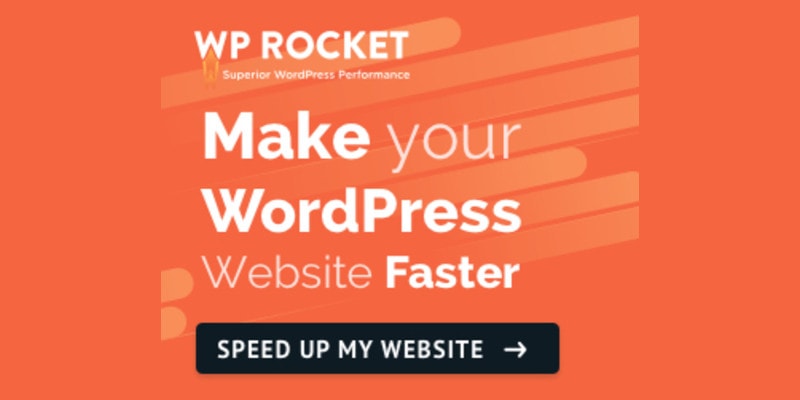This vibrant advertisement features an orange background with striking white text, designed to capture attention. Dominating the large rectangular orange space, the ad prominently displays the message, "WP Rocket Superior WordPress Performance," in clean, bold white font.

A small orange house icon, overlaying one of the vertical orange stripes in the background, adds a touch of character and visually anchors the top of the ad. The text underneath, "Make your WordPress website faster," includes bold, enlarged words for emphasis, drawing the reader’s eye immediately to the key benefits.

Towards the bottom, a black box with white lettering demands action, urging viewers with the call-to-action, "Speed Up My Website," alongside a white forward arrow icon indicating progression and improvement. 

Overall, the image maintains high-quality resolution with no significant blurring or pixelation, ensuring all elements are crisp and professional. The symmetry and centering of both the text and the background stripes provide a balanced and focused composition, making the ad visually appealing and effective in conveying its message.